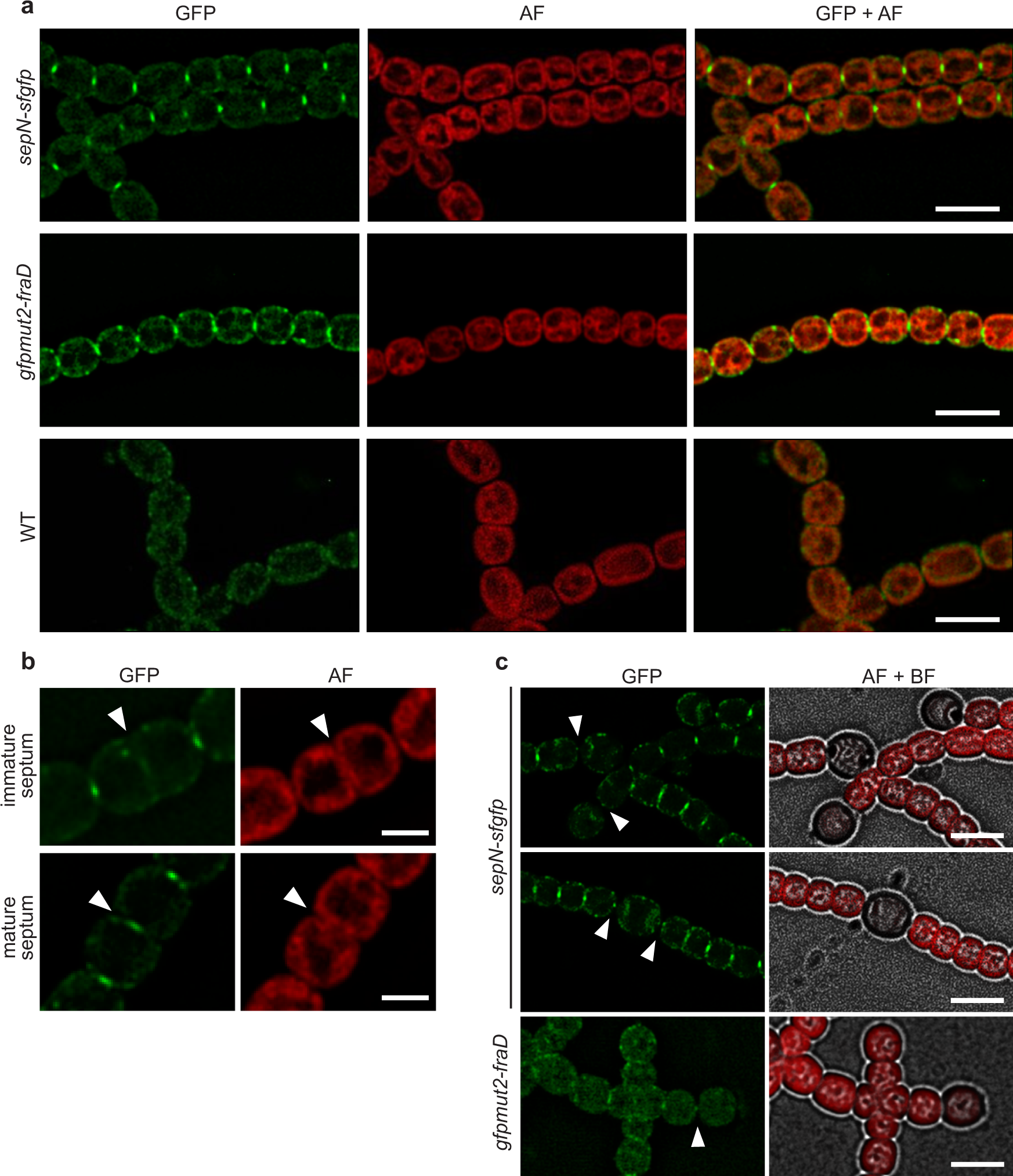The figure presented consists of three main panels labeled A, B, and C. 

Panel A features a grid of nine images arranged in three columns and three rows. The left column shows images stained with green dye, labeled GFP (green fluorescent protein), depicting chains of small ovals or beads. The middle column displays images stained with red dye, labeled AF, forming similar chain patterns in red. The right column shows the overlap of the green and red dyes, resulting in a mixed amber color. These images collectively illustrate various views and compositions of the chain structures.

Panel B, situated below Panel A to the left, contains four images organized in two rows and two columns. The two left images, labeled GFP, show close-up views of the green-stained chains. The right images, labeled AF, offer close-ups of the red-stained chains. White arrows and triangles highlight specific regions such as splits within the chain structures, with labels indicating "immature septum" and "mature septum," suggesting stages of a developmental or structural process.

Panel C, located to the right of Panel B, comprises six images in two columns and three rows. The left column includes images stained with green dye (GFP), while the right column displays a combination of red dye (AF) and additional grayscale imaging techniques. Triangular markers point out particular aspects within these images, emphasizing notable features in the chain formations.

Overall, the figure employs green and red fluorescent dyes to visualize and compare the structural details and developmental stages of chain-like formations, leveraging multiple imaging techniques and annotations for clarity.